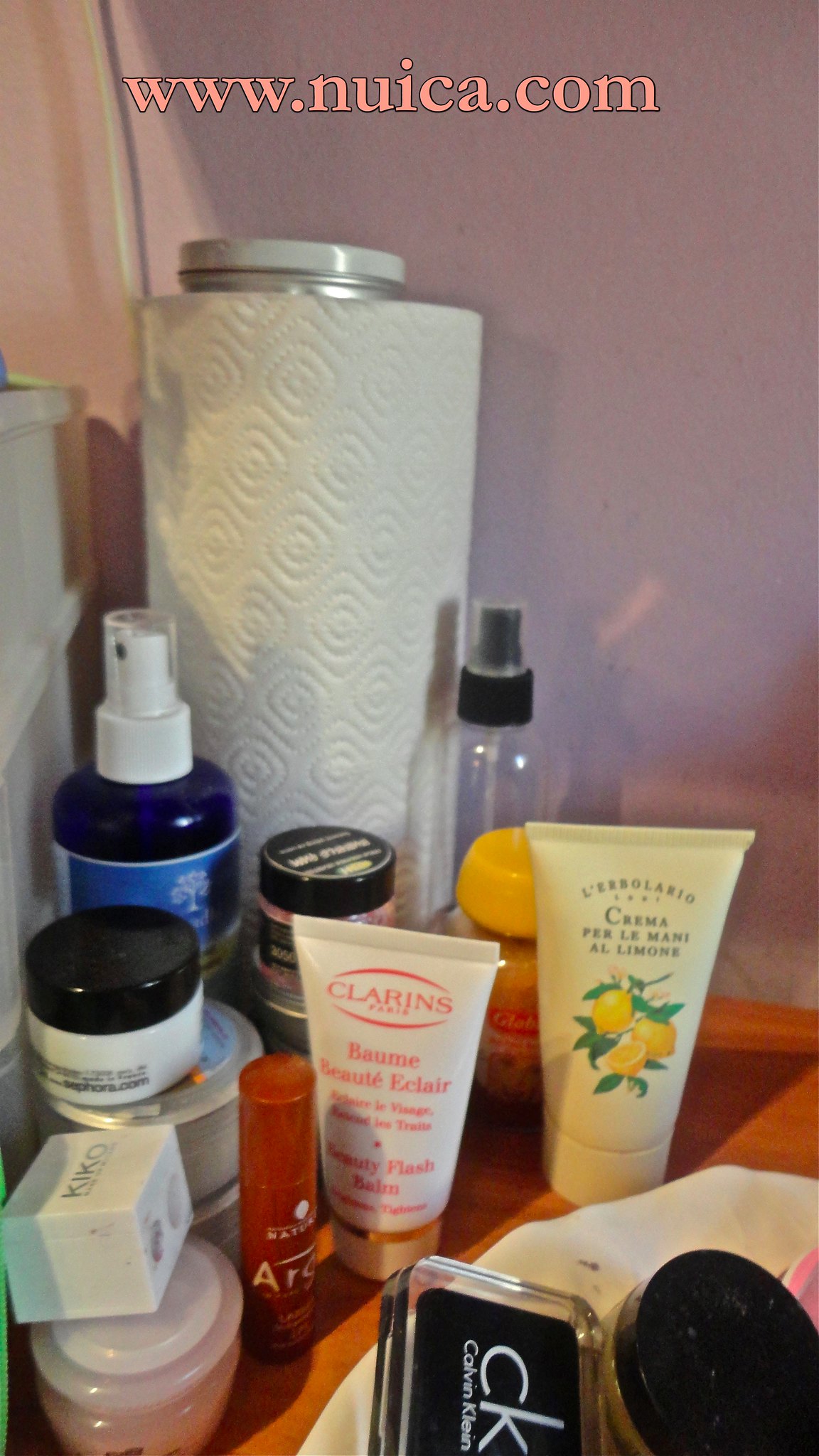This photograph showcases an orange countertop set against a vibrant purple wall. At the top of the photograph, the website "www.nuica.com" is prominently displayed in pink letters. Positioned towards the middle-left corner of the countertop, within a vertical holder, is a roll of paper towels. The countertop is cluttered with various cosmetics and skincare items, neatly arranged on a tray. These include an array of bottles, squirt containers, lotion bottles, and boxes. Among the items, an orange lipstick tube stands out. A detailed inventory reveals items such as a "Beauty Flash Balm" in a pink and white tube, a yellow tube labeled "Crema per la mano al limon" (lemon hand cream), and a large blue squirt bottle positioned at the back. The collection presents a vivid and eclectic mix of beauty products against the colorful background.